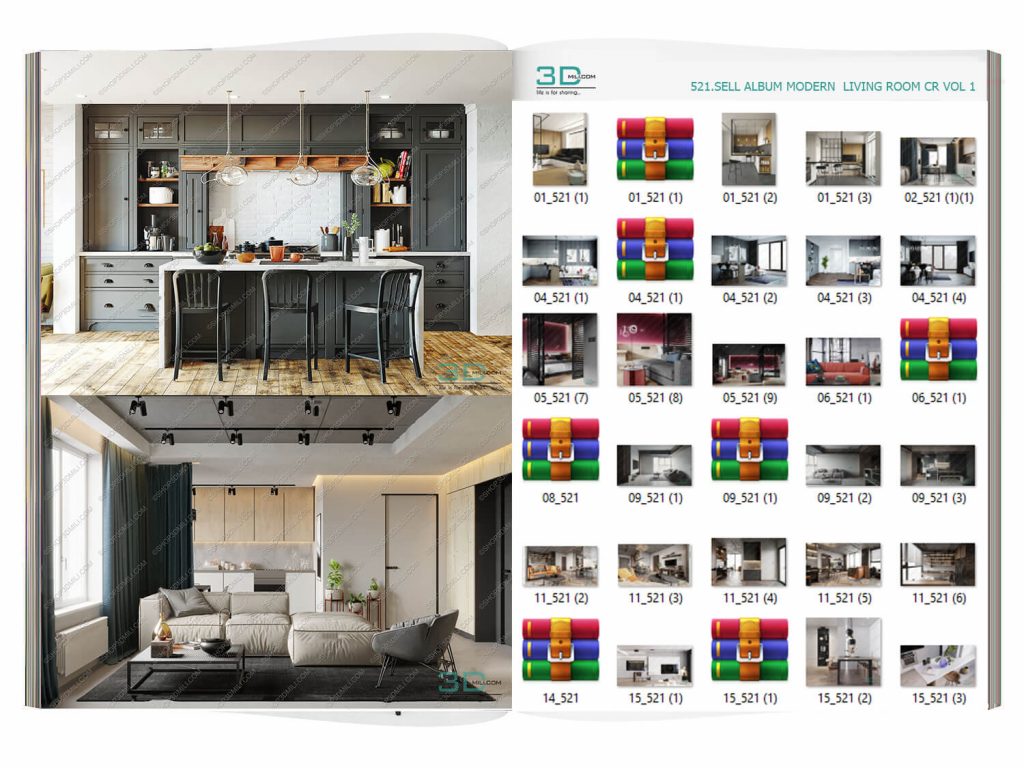The digitally created catalog or magazine displayed in the open book features two distinct photos on the left page: the upper image showcases a modern kitchen space, while the lower image reveals a cozy living room area. On the right page, a logo reading "3D" with smaller accompanying text is positioned at the top left corner. The upper right corner bears the title "521 Cell Album Modern Living Room CR Volume 1." Below the title are numerous image icons, each labeled sequentially with codes like "01_521" and "04_521," depicting various interior scenes. Notably, some image icons feature a symbol of three stacked books bound by a belt, indicating that these images are locked.